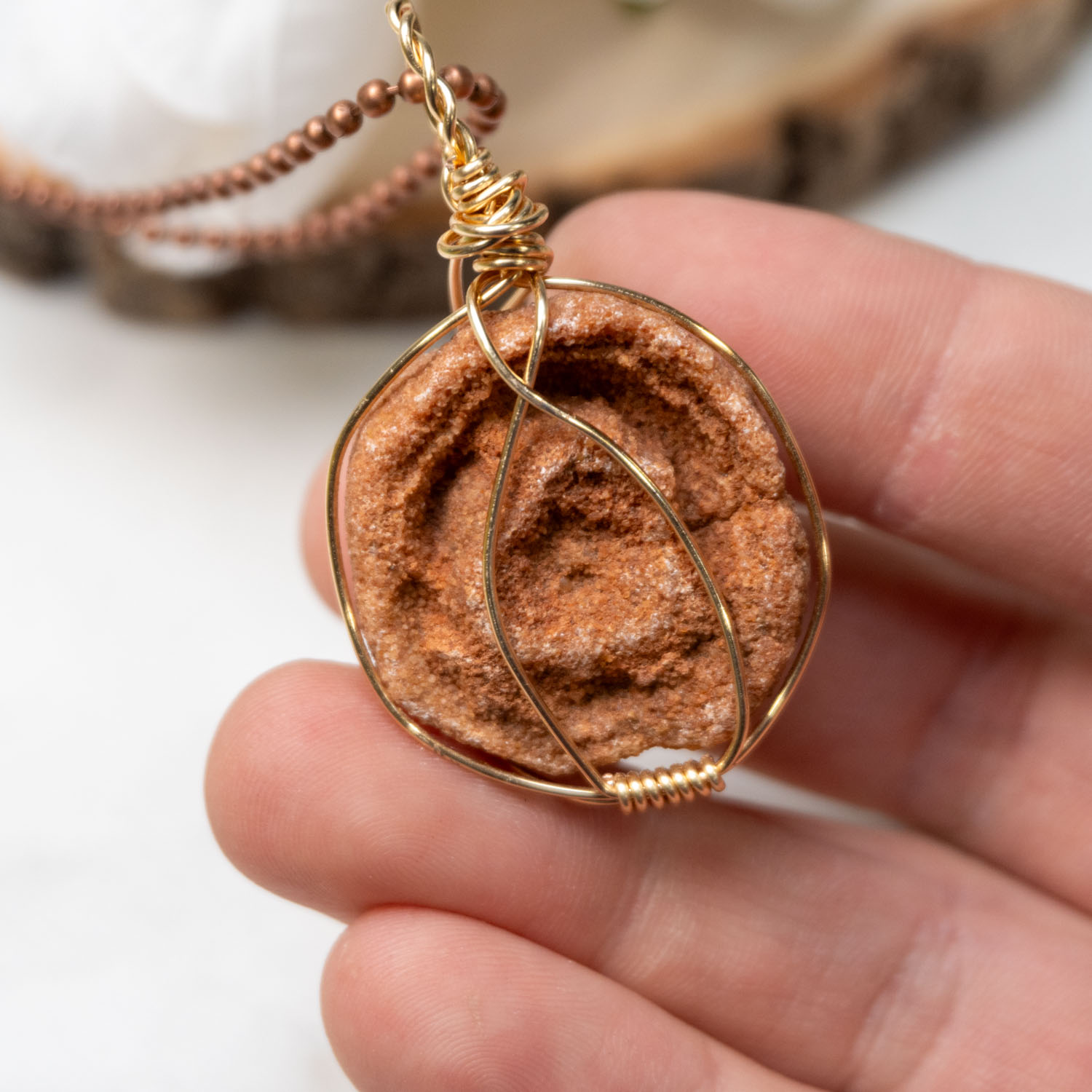The close-up image captures a handmade jewelry piece held by the tips of four fingers from a Caucasian hand. The background is intentionally blurred, highlighting the jewelry against a white backdrop. The main focus is a pendant featuring a roughly textured, brown stone that appears to be handmade or not naturally occurring. This stone is encased in an intricate frame of thin, twisted gold wire, which creates a circular and supportive structure around it. This pendant is attached to a simple chain made of small copper beads. The overall craftsmanship and unique materials lend a rustic yet elegant look to the necklace.